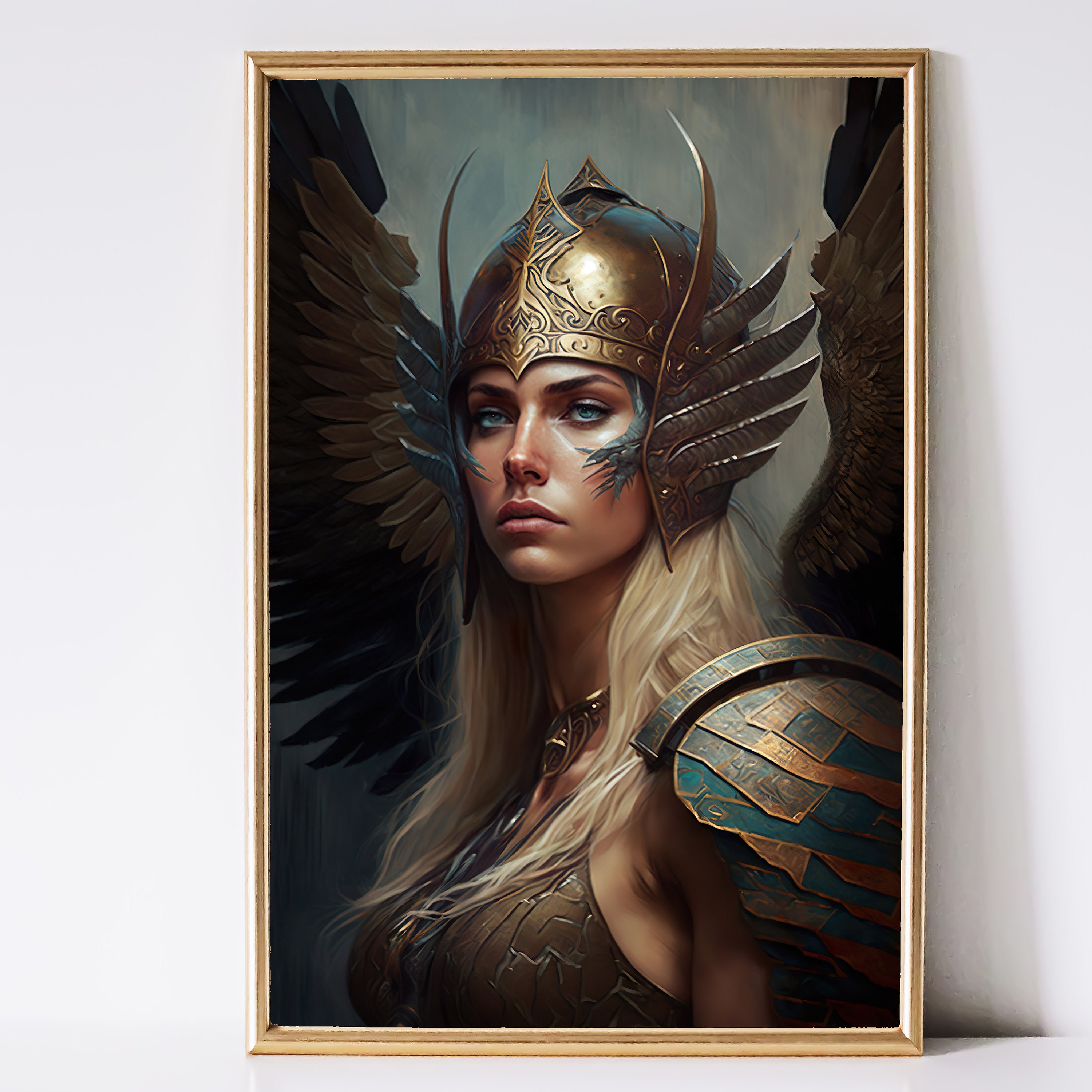The image is a large square photograph featuring a striking piece of framed artwork leaning against a white wall, situated on a white shelf. The frame of the artwork is narrow and gold, adding a touch of elegance to the scene. The artwork itself depicts a fierce young woman dressed as a warrior, with a determined expression on her face. She has long blonde hair that cascades over her shoulders and blue eyes that command attention. The woman is clad in a sleeveless piece of armor that appears to be golden or bronze, and she wears a chain around her neck. Her helmet is adorned with distinctive, curved spikes on each side, adding to her formidable appearance. Behind her, large brown wings are faintly visible, contrasting with the blend of gray and light gray that forms the background, suggestive of a stormy sky. The overall clarity of the image is high, with the bright lighting emphasizing the intricate details of the artwork and its surroundings.